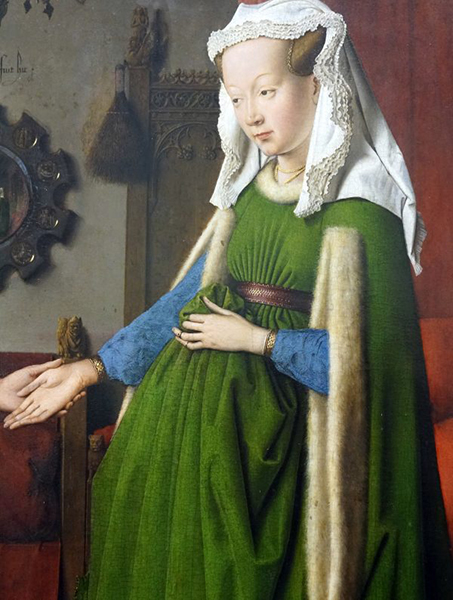In the painting, a woman from the old-world era, reminiscent of times with lords and ladies, stands in profile facing left. She appears to be pregnant, accentuated by her voluminous green robe, which she holds with one hand, causing the fabric to bulge around her stomach. The green robe, worn over a blue dress, features slits through which her arms emerge, and is cinched under her bust with a leather strap. Her head is mostly covered by a white, lacy scarf, revealing only a bit of her brown hair. She extends her right hand outward, where an unseen person holds it gently. She wears a gold necklace and looks pensive. Behind her, the room has dingy walls and features a high-backed, ornately carved chair with a small handheld broom hanging from its corner. Part of an ornate clock is visible to her left, further enriching the historical atmosphere.